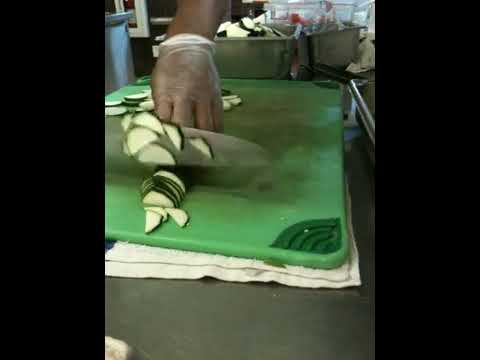In a bustling, professional kitchen, an individual wearing a clear see-through glove can be seen meticulously slicing a cucumber on a green plastic chopping board. The board has rounded corners and a dark green rubber textured pattern. The person is using a sharp silver knife, positioned mid-motion above the vegetable, with several thin cucumber slices clinging to the blade. Numerous neatly pre-cut slices lie to the right of the knife, while the uncut portion of the cucumber remains on the left. The person's gloved hand firmly holds the cucumber in place with fingers curled, ensuring a safe cutting technique. A metal countertop, common in commercial kitchens, serves as the workspace, and silver trays filled with additional cucumber slices are visible in the background. This setup suggests that the individual has been diligently slicing cucumbers for some time.